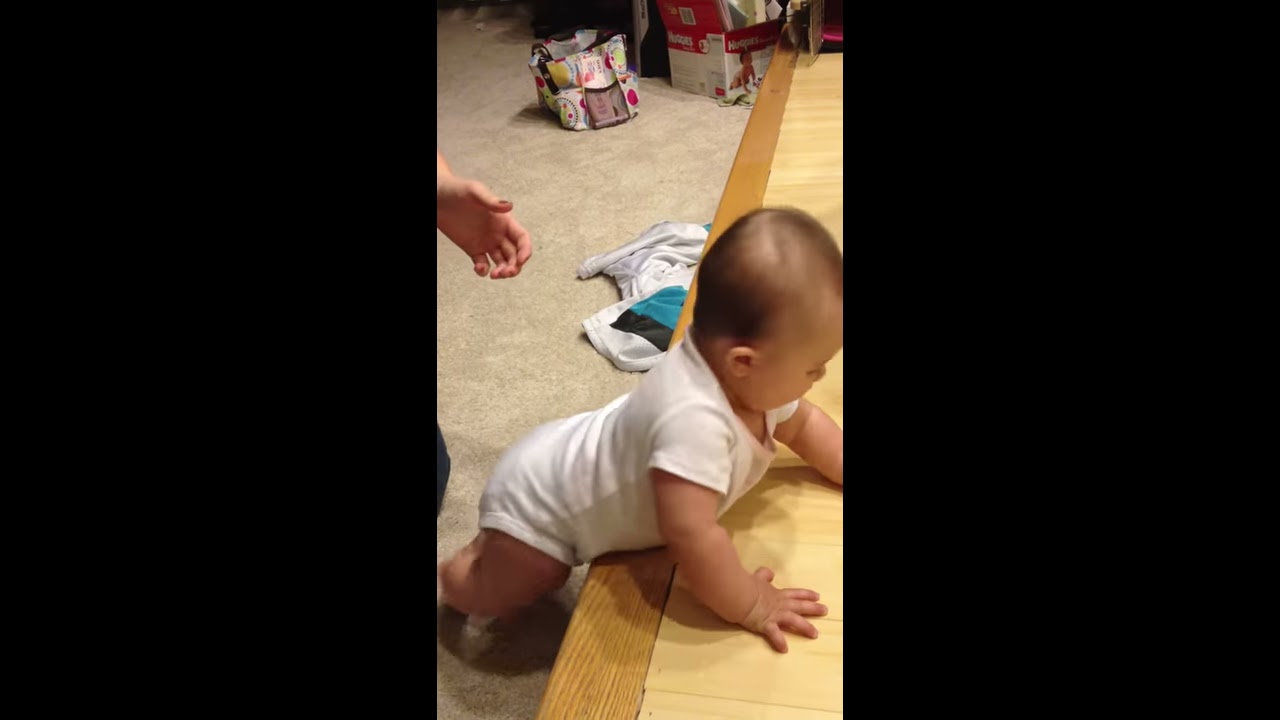This detailed image is divided into three equal panels, flanked on the left and right by black backgrounds. The central panel features a captivating scene of a baby in a semi-crawl position, attempting to propel herself up onto a raised wooden platform. The baby's tiny hands are firmly grasping the edge of the light tan hardwood step that stands out against the surrounding beige carpeted floor. She is dressed in a simple white onesie.

Poised in the background, a deeply attentive figure—presumably the child's mother—extends her left hand from the left side of the image, ready to catch the baby if she loses balance. The mother’s fingernails are visible, though the color is indistinct. Behind the baby, scattered on the floor, is a crumpled blue, white, and black blanket along with some clothing. There is also a travel bag and a conspicuous box of Huggies diapers, signifying a typical domestic environment. The mother's cautious yet ready stance contrasts with the baby's determined effort, capturing a tender moment of care and exploration.